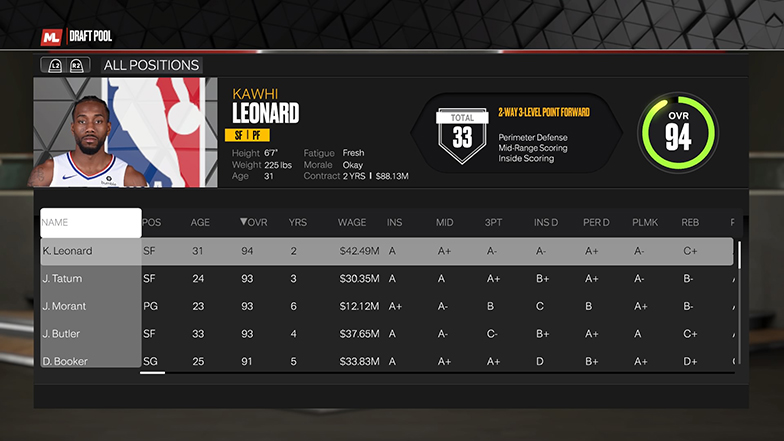The image appears to be a screenshot from a video game, presented on a black background. At the top of the screen, there is an interface that mimics the appearance of a tire. In the top left corner, a section labeled "Draft Pool" is visible. Below this label, a subsection is titled "All Positions" and displays a picture of a basketball player donned in a white jersey.

To the right of the player's image, detailed information about the athlete is provided. The name displayed is Kawhi Leonard, with the following attributes listed: height 6'7", weight 235 pounds, age 31, fatigue status listed as "Fresh," morale indicated as "Okay," and an active contract for 2 years. Additional statistical data includes a total score of 33 and an overall rating (OV) of 94.

Beneath this information, a comprehensive chart is presented, listing the names of various players. The chart details each player's position, age, years of experience, wage, and ratings for different skills including MID (mid-range shooting), 3PT (three-point shooting), INS (inside scoring), PERD (perimeter defense), PLMK (playmaking), and REB (rebounding). The chart is fully populated with data for each player listed.